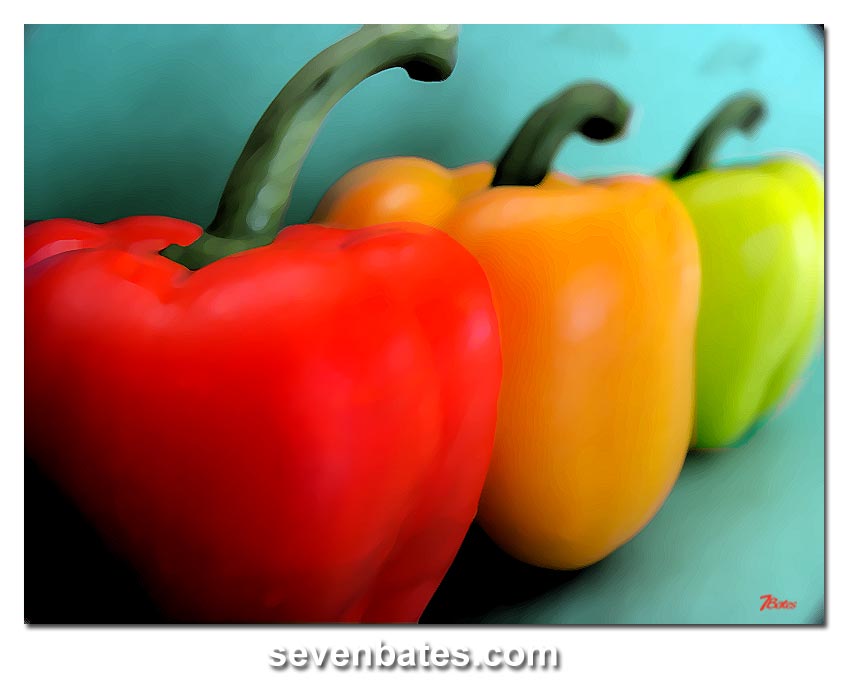This close-up image features three bell peppers in vivid colors—red, orange, and green—arranged in a diagonal line from left to right. The peppers have dark green stems, and their blurred, painted-like appearance suggests an AI-generated image or an oil painting with colors softly merging together. The leftmost pepper, bright red and dominant in size, casts dramatic shadows at the bottom left, while the middle orange pepper is more square and slightly taller. The green pepper on the far right is noticeably smaller and more blurred. The background is a gradient of light bluish-aqua with shadows indicating a light source from the upper right corner. In the bottom right corner of the image, "Bates" is subtly signed in red. Below the image, on a white background with a black border, "7bates.com" is written in white font. Despite the soft focus, the contrasting colors of the red, orange, and green peppers dominate the visual experience.